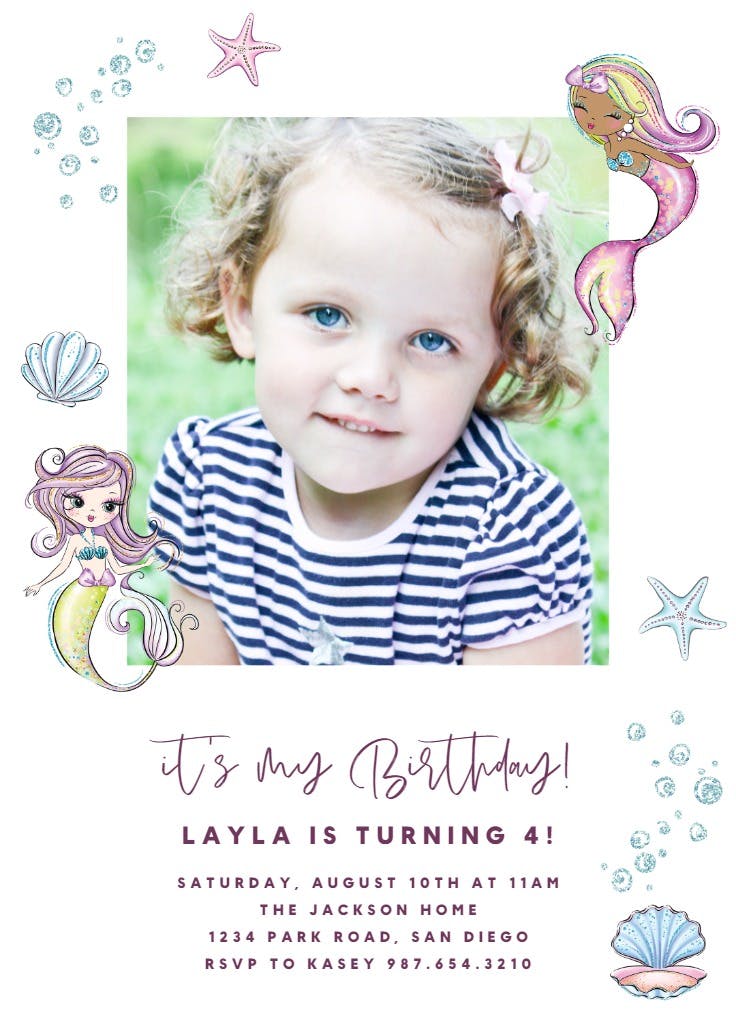This image is a colorful flyer inviting guests to a child's birthday party. Centrally placed, slightly towards the upper middle, is a photo of Layla, a 4-year-old girl with blonde curly hair, wearing a blue and white striped short-sleeved shirt adorned with a small pink bow in her hair. She smiles at the camera with her blue eyes. Below her photo, the text reads, "It's my birthday, Layla is turning four." The invitation details are clearly outlined: "Saturday, August 10th at 11 a.m. at the Jackson home, 1234 Park Road, San Diego. RSVP to Casey at 987-654-3210." The background of the invitation is predominantly white, framed by a thick white border decorated with underwater-themed graphics like seashells, starfish, and bubbles. Additional charm is added by cute, cartoony mermaids—one with pink hair and the other with blonde and pink hair—placed around the photo in the bottom left and top right-hand corners. The text on the flyer is in purple, harmonizing with the mermaid and shell graphics in shades of purple and blue.